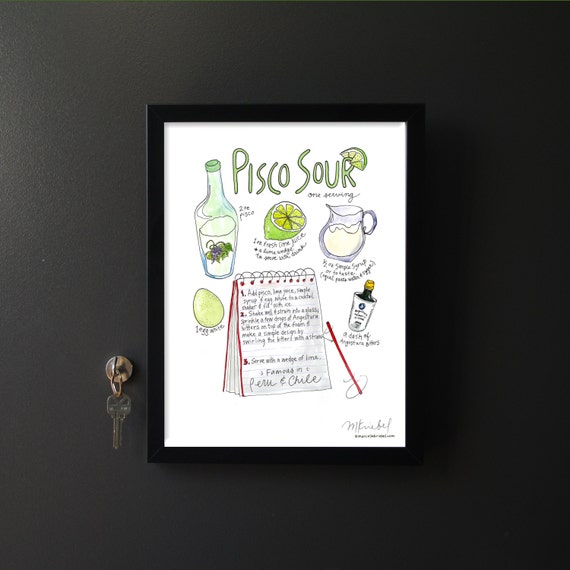The image is a photograph of a hand-drawn illustration within a vertically oriented, brown wooden frame, mounted on a black wall. The framed illustration depicts the recipe and ingredients for making a Pisco Sour beverage, prominently featuring a spiral-bound notebook on a white page. The notebook, outlined in black with a red edge and a red pen beside it, lists the steps numbered 1, 2, and 3, though the text is slightly blurred. The handwritten green title "Pisco Sour" with an underlined "R" appears at the top, and below the instructions, it is noted as "famous in Peru and Chile." The illustration includes various ingredients such as a bottle of Pisco, a cut lime, an egg, a pitcher (implying simple syrup), and a small bottle of bitters, all clearly drawn around the notebook. On the left side of the photograph, a key hangs from a metal key hook affixed to the wall, adding an interesting detail to the scene. The overall setting is bright with plenty of lighting, highlighting the clarity and detail of the illustration.